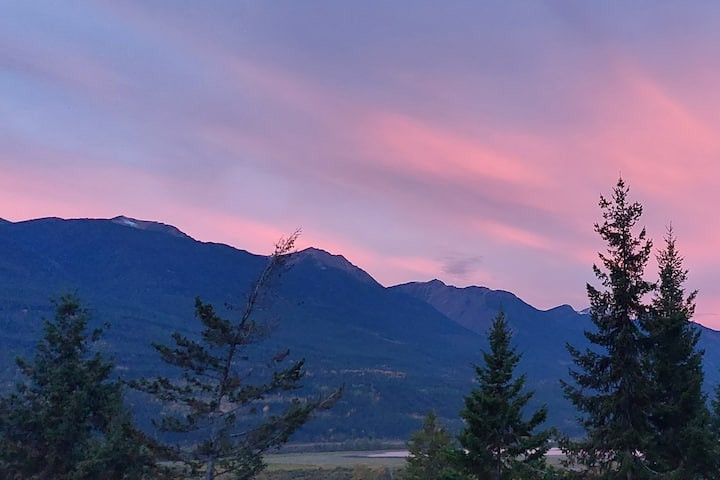The image depicts a serene natural landscape captured in a wide vertical rectangular format. In the foreground, conical-shaped pine trees with dark green foliage frame the scene in the bottom right and left corners. These trees partially obscure a vast, lush green field that extends into the middle distance. The field is dotted with what appears to be a silver, flat lake, adding a reflective element to the scene.

Beyond the field, a majestic mountain range dominates the background. The mountain range, rendered in dark bluish-gray tones, stretches across the width of the image, appearing taller and more jagged on the left side before angling downwards towards the right. This rugged terrain is capped with rocky, uneven peaks.

Above the mountains, the sky showcases a stunning gradient of colors, likely captured during the evening. Shades of light blue blend seamlessly with delicate hues of pink, orange, and white, reminiscent of a cotton candy sky. Faint, wispy clouds stretch across the upper part of the image, adding texture and depth to the tranquil backdrop. This setting vividly captures the beauty of a peaceful, scenic location at dusk, with natural elements harmoniously blending together to create a picturesque view.